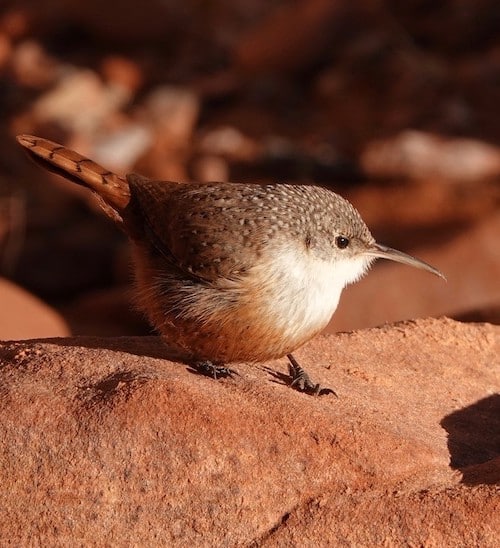The image features a small, round bird perched on a porous, grayish-brown rock, which could be part of a stone wall. The bird stands out in sharp detail against a blurred background, which hints at a natural, perhaps desert-like setting. The background is so out of focus that identifying specific elements, whether rocks or nature, is impossible. The bird, facing slightly to the right, boasts a fat, round body with a large belly, characterized by white patches below its chin and on the upper part of its chest, transitioning to a reddish-brown underneath. It has a long, sharp beak and small wings, complemented by a long, stripe-patterned tail. Its top feathers are a mix of browns, blacks, and creams. The photograph is high-quality, likely taken by an adept nature photographer, capturing the bird in a vivid, life-like pose. There are no other animals or text in the image, which might be suitable for an educational book or nature portfolio.